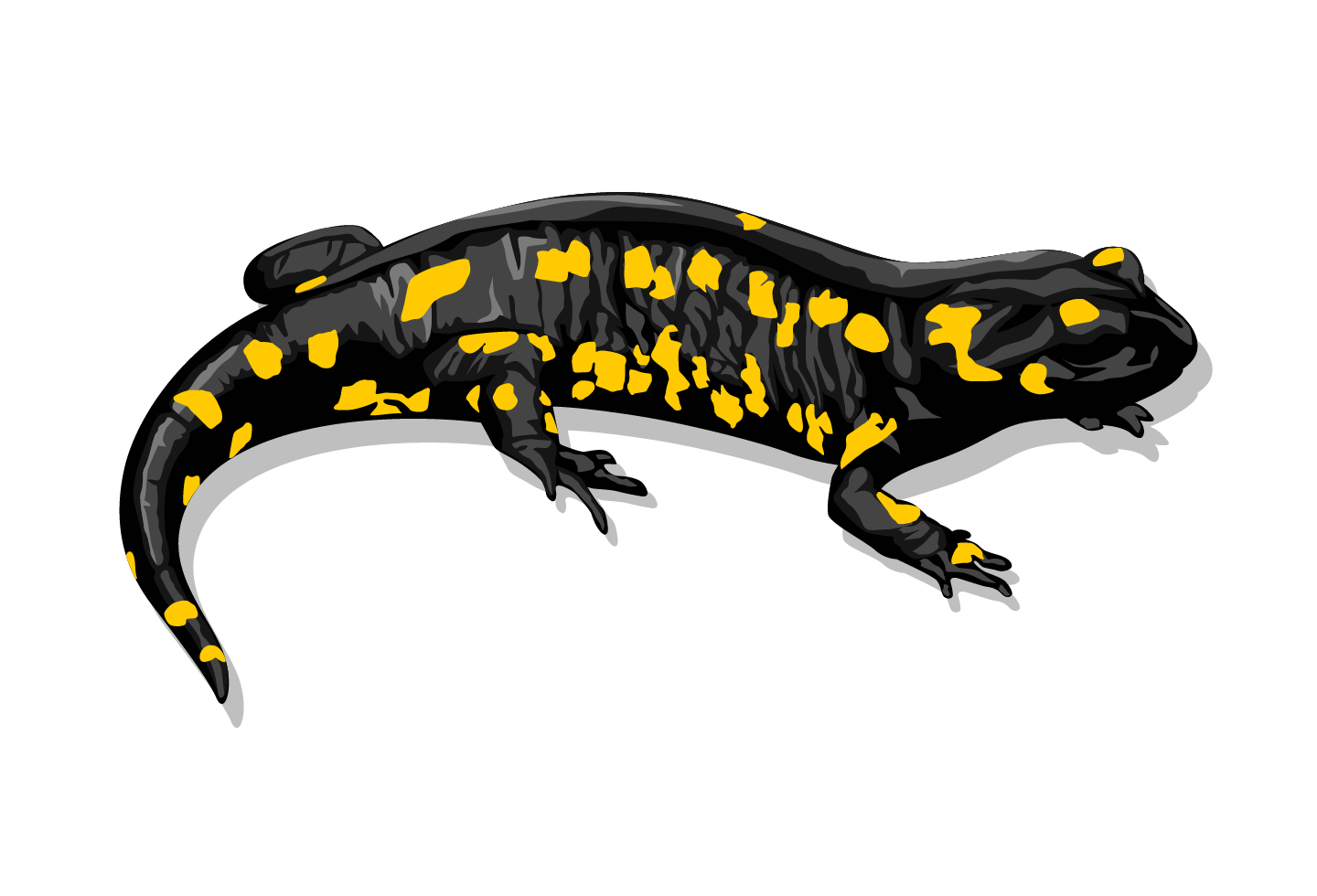This is a detailed illustration of a black reptile, possibly an iguana or salamander, displayed in a side view on a white backdrop with lighting from above, casting a shadow beneath it. The creature features a medium-length tail positioned to the left and a head to the right. The animal's skin is primarily dark black with irregular yellow or orangey-yellow splotches covering its head, back, sides, legs, and feet. Additionally, there are lighter gray areas forming a splotchy stripe pattern along its back. Three feet and four short, slumpy legs are visible, with each foot having well-defined fingers and small nails. The eyes are not well-defined, appearing to be very dark, likely black, and the mouth is closed, revealing no tongue. The illustration employs detailed shading to enhance its realistic appearance, giving the creature a shiny, well-colored look.